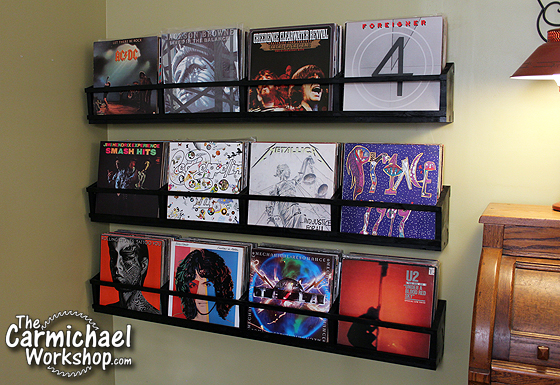The image depicts the interior of the Carmichael Workshop, identified by the text "the Carmichael Workshop" superimposed in the lower left corner. Prominently displayed on the left side and middle of the image are three rows of black shelves mounted on a white wall, each holding four different LP album covers for a total of twelve albums. Notable album covers include those from bands like Foreigner, U2, Deep Purple, and ACDC. Directly adjacent to the albums on the right side is part of a vintage brown roll-top desk, adding a nostalgic touch to the ambiance. Above the desk in the upper right corner, there appears to be a copper-shaded light fixture, casting a warm glow in the scene. The detailed arrangement and classic furniture give the workshop a cozy, retro vibe.